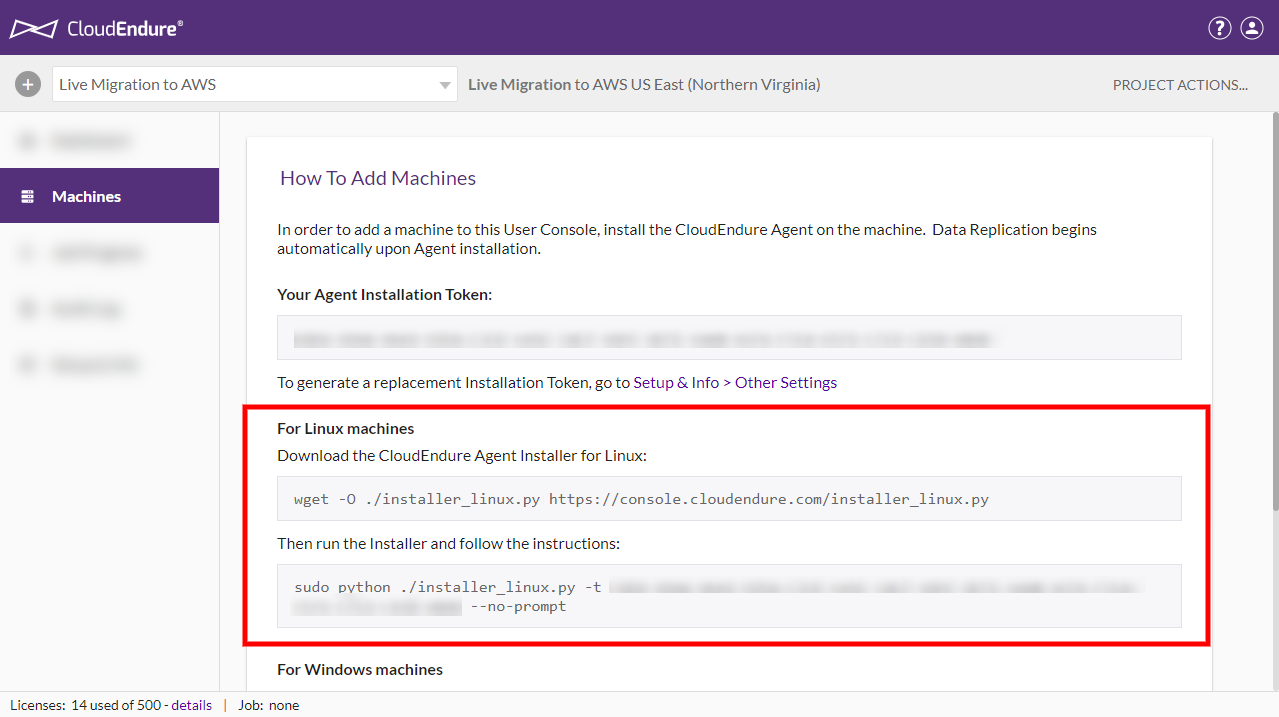At the top of the image, there is a dark purple border with the text "CloudEndure". To the left of this text, two side-lying triangles with their tips facing each other create a bow tie-like pattern. On the far right side of the top section, there is a circle with a question mark inside it and another circle containing a generic profile picture. Below this, a light gray area is visible, featuring a dark gray circle on the left with a plus sign in the middle. Here, a drop-down menu displays "Live Migration to AWS". To the right, it extends to read "Live Migration to AWS US East (Northern Virginia)" and further right, it displays "Project Actions...". Beneath this section, a large white box dominates the image. At the top of this box, the text "How to Add Machines" is prominently displayed. Below this, smaller text reads: "In order to add a machine to this user console, install the CloudEndure agent on this machine. After that, replication begins automatically upon agent installation." Toward the bottom is the instruction "Your agent installation token." Directly under this, there is a rectangular box that has been deliberately blurred out, obscuring the contents.